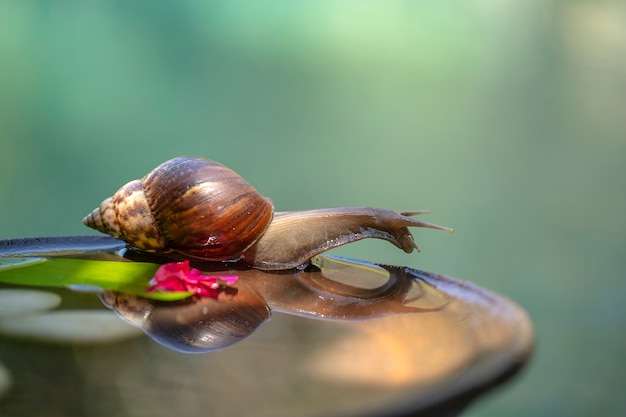This realistic, close-up nature photograph captures a snail slowly moving across a shiny, reflective surface, likely a wet rock or metal. The surface is round, brown, and glossy, casting a mirror-like reflection of the snail underneath it. The snail, with a light tan and brown body, sports a brown shell splotched with white on its back-left side. It has two extended antennae and a smaller one on its head, reaching forward as if inspecting its environment. To the left of the snail, there’s a small green leaf accompanied by a red object, possibly a flower or shiny paper. The background out of focus, presents a soft, muted blend of green and gray tones, suggesting an outdoor setting or a well-lit studio, emphasizing the snail as the central focus of the image.